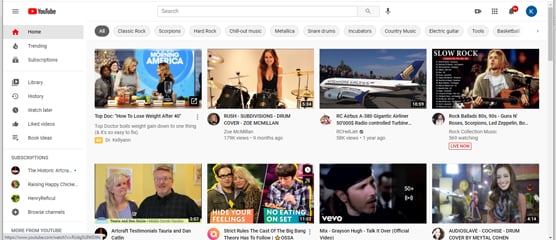In this screenshot, set against a white background, we see a page from the YouTube website. Though the image is quite blurry, some details are discernible. At the top, there's a white header featuring the YouTube icon in the upper left corner, a red square with a white play button, accompanied by "YouTube" in bold black letters. Centrally located on the top header is a white search bar, and in the upper right corner, a blue circle with a white "K" indicates the user avatar. Adjacent to this, the notifications icon and battery icon are visible.

Just below the header are the category menu buttons, ranging from left to right: All, Classic Rock, Scorpions, Hard Rock, Chill Out Music, Metallica, Drums, Incubators, Country Music, Electric Guitar, Tools, and Basketball.

Beneath these categories, several video thumbnails are partially visible. In the top left corner, there's an image showing the host from Good Morning America standing in front of a table. To its right, a video features a young woman sitting at a drum set with the title, "Drum Cover Zoe McMillan." Further to the right is a thumbnail of an airplane on a runway, titled "RC Airbus." Lastly, an image of Kurt Cobain holding a guitar fills the screen's bottom right corner, with "Slow Rock" displayed in white text.